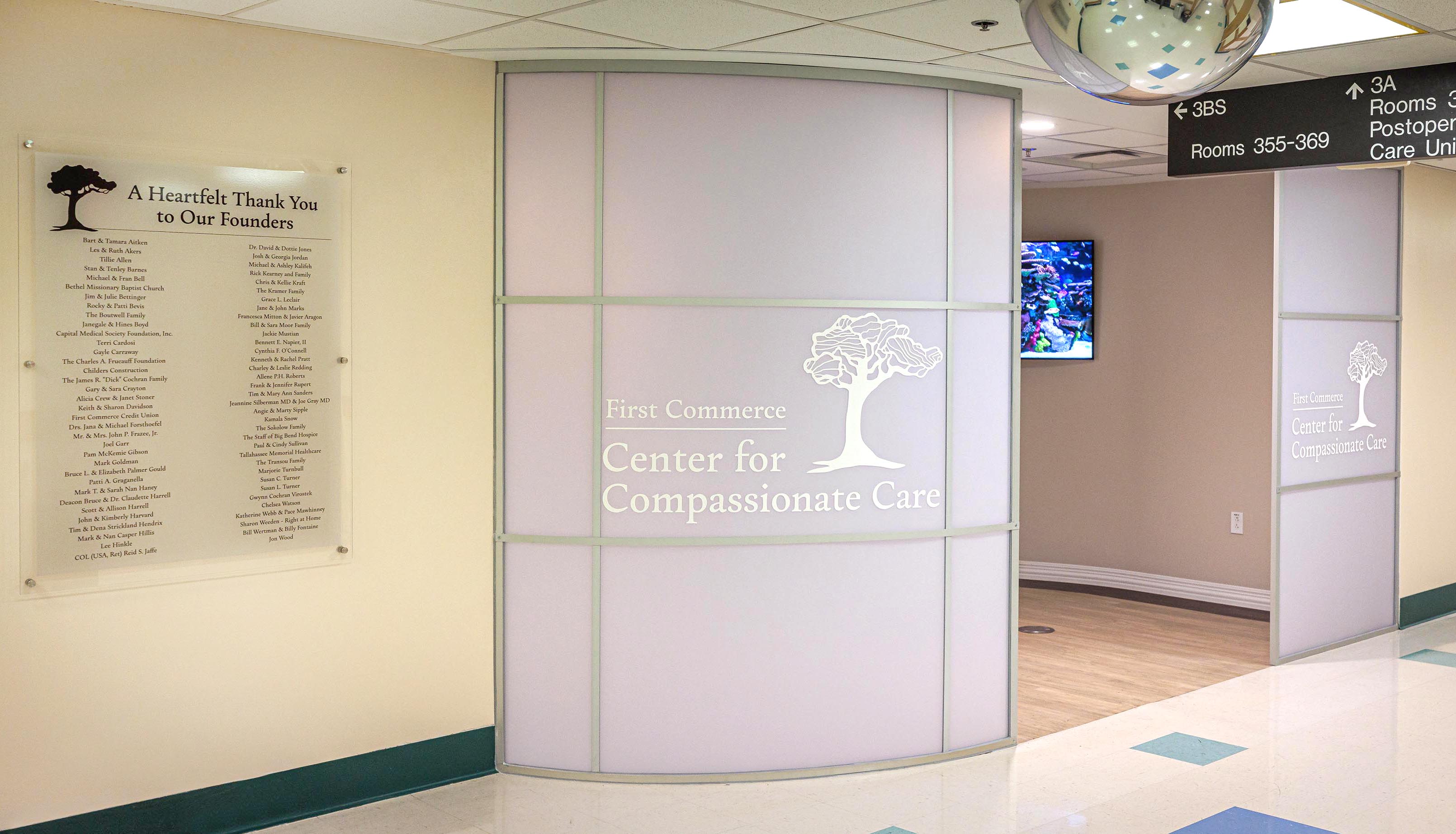This detailed, horizontally oriented photograph depicts the interior of a hospital or care facility. Prominently featured is a ceiling-mounted mirror ball next to a sign directing patients and visitors. The sign indicates that "3BS" with rooms 355 to 369 is to the left, while "3A" with the post-operative care unit lies straight ahead. Below this directional sign is an entryway that serves as a focal point. Above the entryway, illuminated letters inscribed on a translucent, milky gray wall read "First Commerce Center for Compassionate Care," accompanied by an image of a tree.

To the left of the entryway, a light yellow wall displays a plaque which expresses "A Heartfelt Thank You to Our Founders," listing numerous names in gratitude. Inside the entryway, a part of a video screen can be glimpsed on the wall. The entryway's floor consists of white tiles interspersed with blue squares, while transitioning toward 3BS, the flooring changes to a wood grain pattern. The layout and signage provide clear navigation, enhancing the welcoming atmosphere of the care facility.